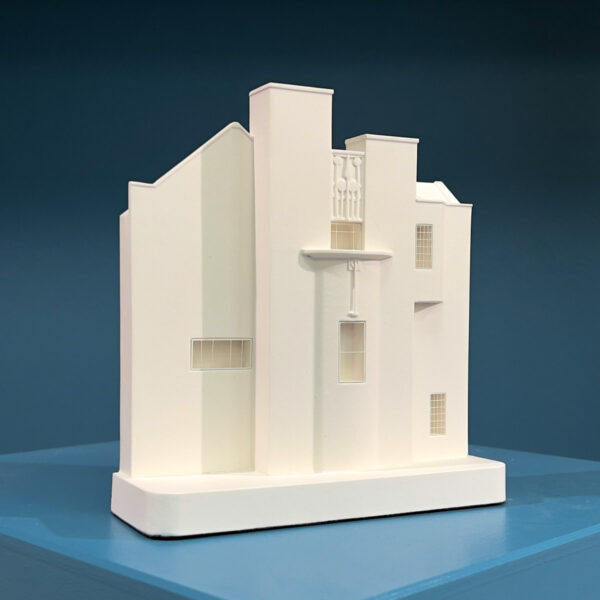The photograph showcases a three-dimensional model of a rather tall, tan-colored house with intricate architectural details, set against a dark blue background that fades to a grayish hue at the top. The background appears bluish-teal, contributing to the image's overall aesthetic. The model sits on a blue, diamond-shaped table, which is tilted slightly, affecting the perspective. The house features a pointed, triangular roof on the left, and sports multiple windows: one centrally placed on the lower level, directly above it another one, and two on the right side—one on the upper floor and another on the lower floor. Additionally, there's a middle window on the left side. The structure is accented by two prominent white chimneys that project light gray shadows, adding depth to the model. Despite its detailed design, the front of the building oddly lacks any visible doors. The white color of the model contrasts subtly with the cream hues and shadows cast upon it, enhancing the intricacy of this architectural representation against its serene background.